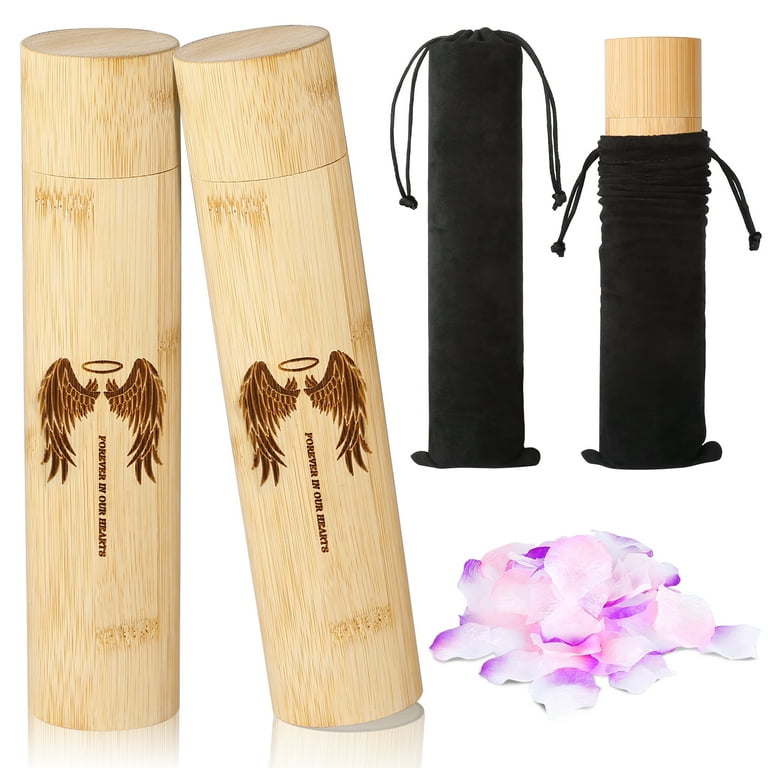The image features four cylindrical wooden memorial objects, two prominently displayed in the foreground with the words "Forever in Our Hearts" engraved alongside an image of angel wings and a halo. The cylinders, light brown and appearing to have removable caps, are likely commemorative items for someone who has passed away, intended as keepsakes for loved ones. The cylinder on the right is leaning against the one on the left. In the background, one cylinder is fully enclosed in a black carry-on bag with drawstrings, and another cylinder's top is visible, suggesting it is partially encased. A tropical floral design with pink, light pink, white, and purple petals is present in the bottom right corner, adding a sentimental touch to the scene.